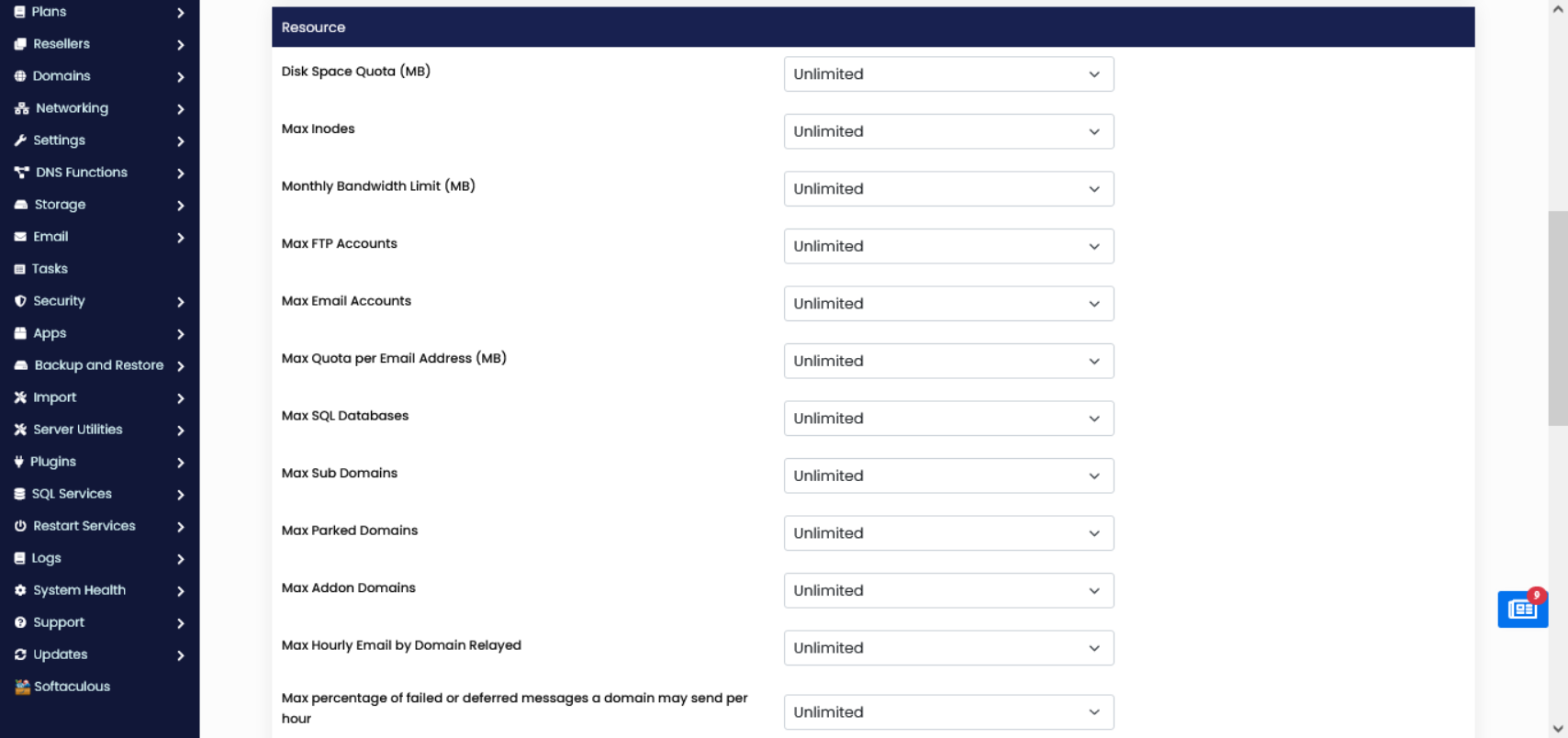This is a detailed screenshot of a web page displaying a computer management dashboard. 

On the left side, a vertical list of options is presented against a dark blue background with white text. The list includes: 
- Plans
- Resellers
- Domains
- Networking
- Settings
- DNS Functions
- Storage
- Email
- Tasks
- Security
- Apps
- Backup and Restore
- Import
- Server Utilities
- Plugins
- SQL Services
- Restart Services
- Logs
- System Health
- Support
- Updates
- Softaculous

Adjacently on the right, the larger, main area of the dashboard has a white background with a blue header labeled "Resources." Below this header, there is a list with black text, detailing various resource categories:
- Disk Space (Quota in MB)
- Monthly Bandwidth Limit (MB)
- Max FTP Accounts
- Max Email Accounts
- Quota per Email (MB)
- Max SQL Databases
- Max Subdomains
- Max Parked Domains
- Max Add-On Domains
- Max Hourly Emails by Domain (Relayed)
- Max Percentage of Failed or Deferred Messages a Domain May Send per Hour

Next to each of these resource categories, there is a dropdown menu, each currently set to "Unlimited," allowing for adjustments to these limits.